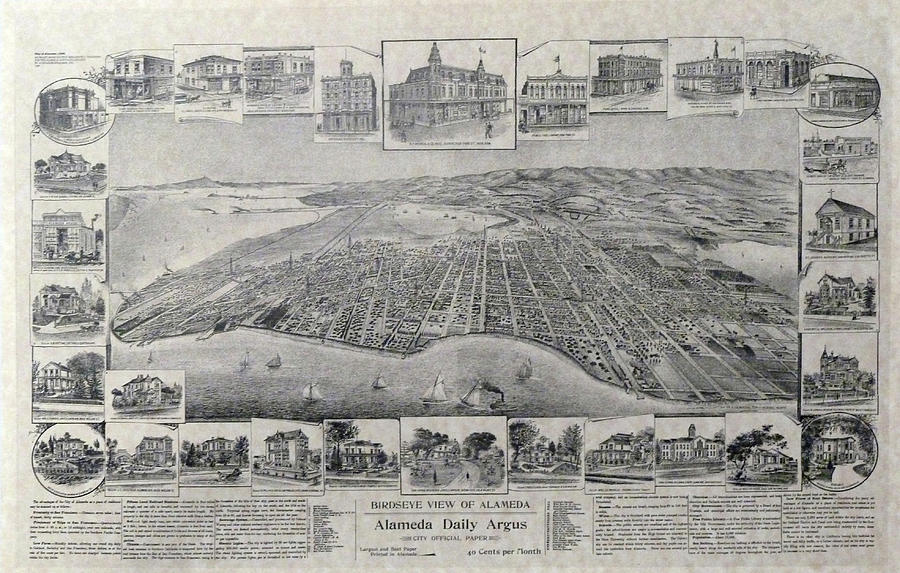This black and white vintage bird's eye view map, likely from the late 1800s or early 1900s, showcases the initial stages of city development in Alameda. The central illustration vividly captures the expanse of the budding city with a picturesque waterway in the foreground, dotted with sailboats. Encircling the main image, a detailed border features various buildings and landmarks specific to Alameda, each meticulously drawn to highlight their significance. The bottom section of the map bears tiny, almost unreadable text with the prominent title, "Bird's Eye View of Alameda, Alameda Daily Argus, City's Official Paper, 40 cents." The entire composition is rendered on high-quality, thick cotton paper, indicative of the prestigious presentation and preservation of this historical document.